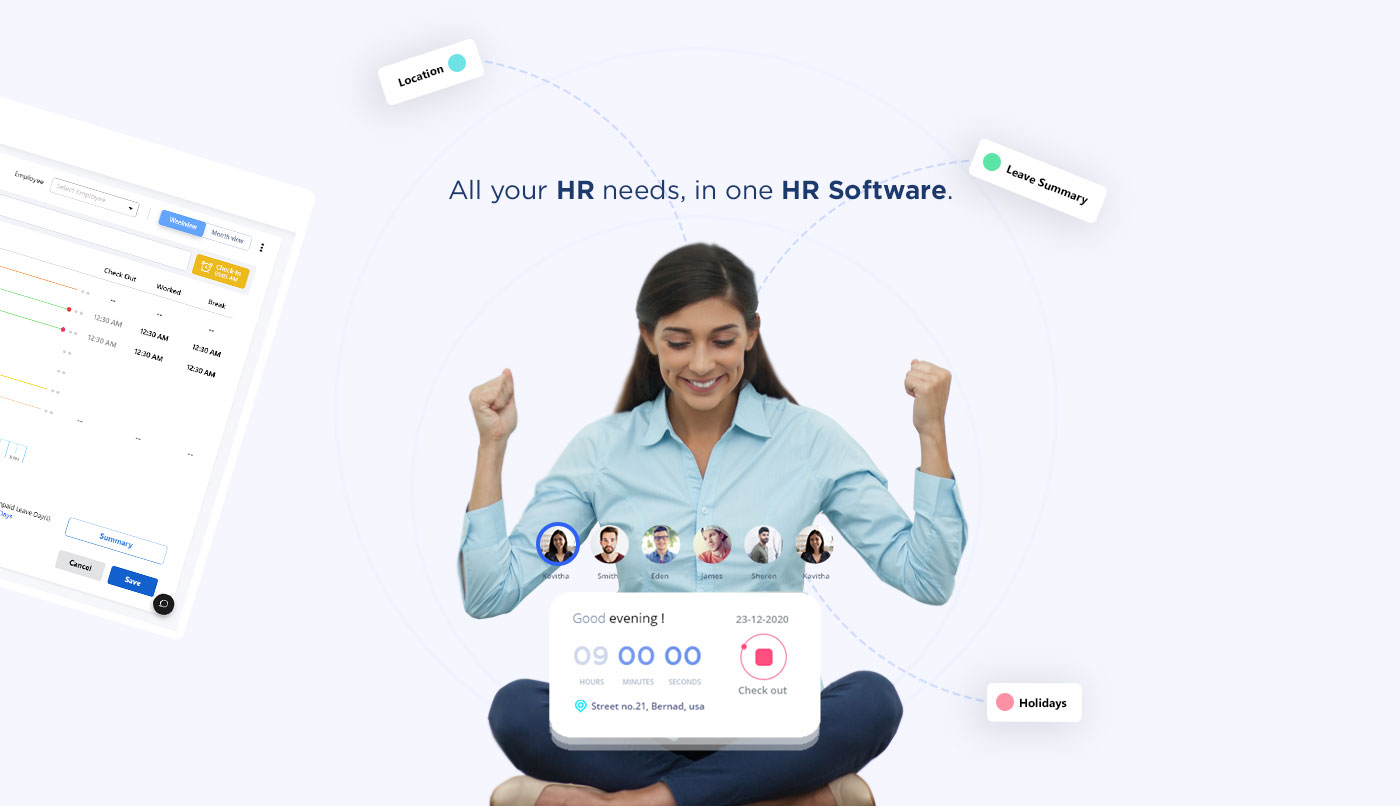A screenshot of a website features a woman sitting cross-legged, exuding joy and success. She is dressed in a light blue, long-sleeved button-up shirt and dark blue pants, paired with beige platform slippers or closed ballerina shoes. The woman has long brown hair tucked behind her ears and is smiling broadly, with her downcast eyes showcasing her visible teeth. Both of her fists are clenched and raised in triumph. Above her, in blue lettering, the text reads, "All your HR needs in one HR software." Surrounding her head are floating tags with words like "location," "leave summary," and "holidays." Beneath this imagery, a section of the screen displays "Good evening," followed by the current date and a stop button for checking out.